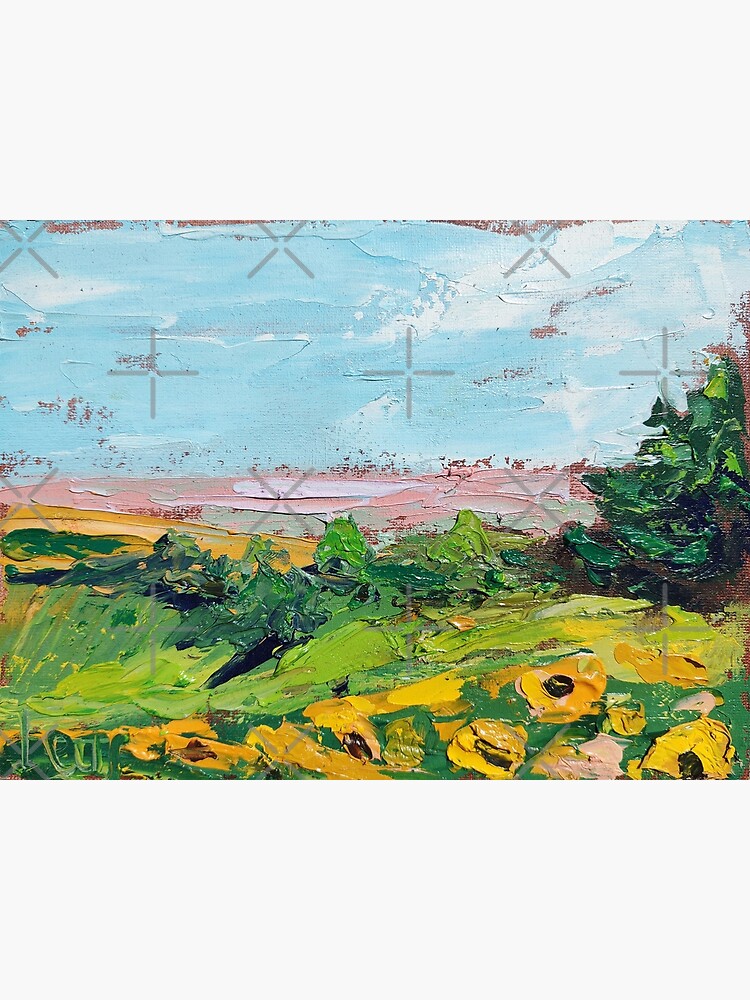This image is a highly textured, abstract oil painting depicting a vibrant natural scene. The foreground features an expanse of rolling green hills dotted with thick, expressive brushstrokes of blue, green, and yellow paint. These hills are embellished with clusters of tall pine trees on either side, smaller green bushes, and a scattering of yellow flowers with dark brown centers, possibly resembling sunflowers. The painting's heavy use of paint creates a three-dimensional effect, with chunky strokes that seem almost touchable.

Above the hills stretches a horizontal swathe of pink, representing an indistinct, abstract layer that gives way to the sky. The sky itself is a soft light blue, interspersed with thick, white brushstrokes suggesting clouds. The application of paint throughout the scene varies in thickness and technique, offering a tactile, layered appearance that enhances the painting's depth and texture.

Adding an unusual element to the artwork, the entire image is overlaid with transparent layers forming plus and cross shapes, which are somewhat distracting but add to the abstract nature of the piece. Despite its abstraction and lack of detailed realism, this oil painting invites various interpretations and evokes a vivid, dynamic portrayal of nature.